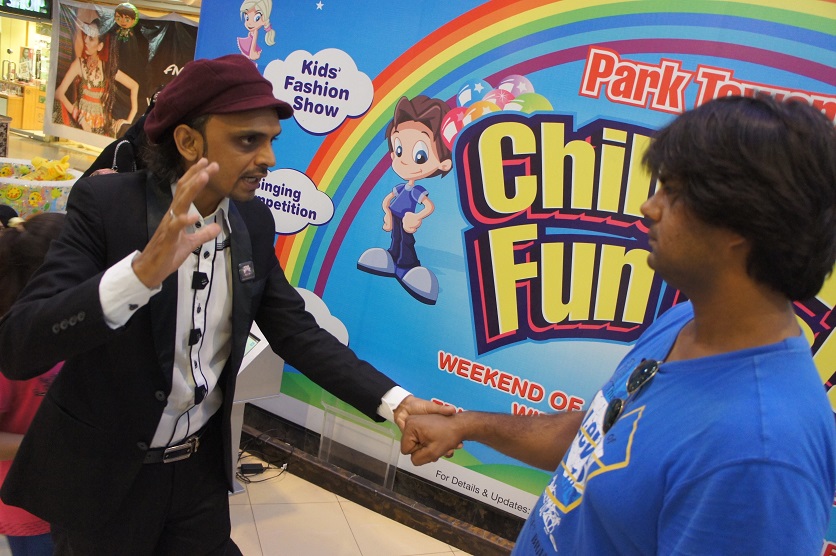In this photograph, two South Asian men are facing each other in a setting that features a vibrant and whimsical backdrop. The man on the right is wearing a blue Levi's t-shirt, with dark-colored lenses on silver-framed sunglasses clipped to his collar around his neck. He has long, plentiful dark hair and is holding the hand of the man opposite him. The man on the left, dressed in a black suit over a white shirt, accessorizes his outfit with a maroon beret cap. Both men display serious expressions as they interact. The background is striking, presenting a colorful rainbow that transitions through red, orange, yellow, green, dark blue, light blue, and purple hues. It is part of a poster that reads "Kid's Fashion Show Imagining Competition," adorned with cartoon images of children. The floor beneath them is white, and the setting appears to be in a mall, adding to the intriguing contrast between the playful backdrop and the serious interaction of the men.